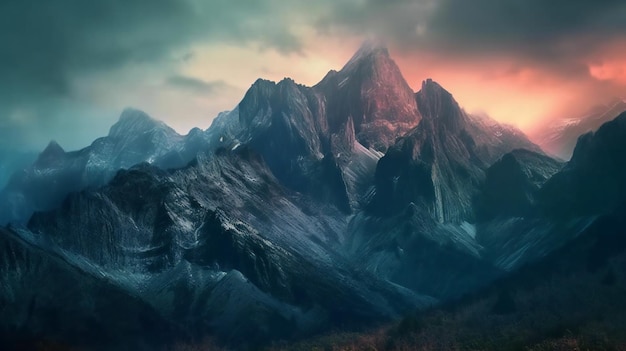The image is a horizontally rectangular, AI-generated artwork, approximately four inches wide and two inches high. It features a striking mountain scene where the aesthetic blends photorealistic and computer-generated elements. The central focus is a large, jagged, rocky mountain that dominates the canvas, with its peak reaching into a dramatic sky filled with clouds.

In the foreground, to the lower right, a hillside colored in dark blue-gray tones slopes upwards before angling back down toward the bottom center of the image. This hillside is detailed with lines indicating sparse grasses and dark spots representing trees. On the left-hand side, another hill slopes upward, then downward, before rising again towards a smaller peak.

The center of the painting showcases the massive, ominous mountain. The left side of this mountain is tinted in cool blues and grays, while the right side contrasts with warm reds and grays. The background sky is split between a blue hue on the left with dark blue clouds and a vivid reddish-orange on the right, creating a twilight effect. Dark gray clouds hover above, enhancing the scene's dramatic atmosphere. The entire image evokes a sense of dusk, with the orange and yellow glow of a setting sun illuminating the rugged landscape, juxtaposed against the hazy, bluish-green sky on the left. The overall composition conveys a sense of depth and stark beauty with a blend of pastel-like colors reminiscent of cinematic art from movies like "Godzilla vs. Kong."